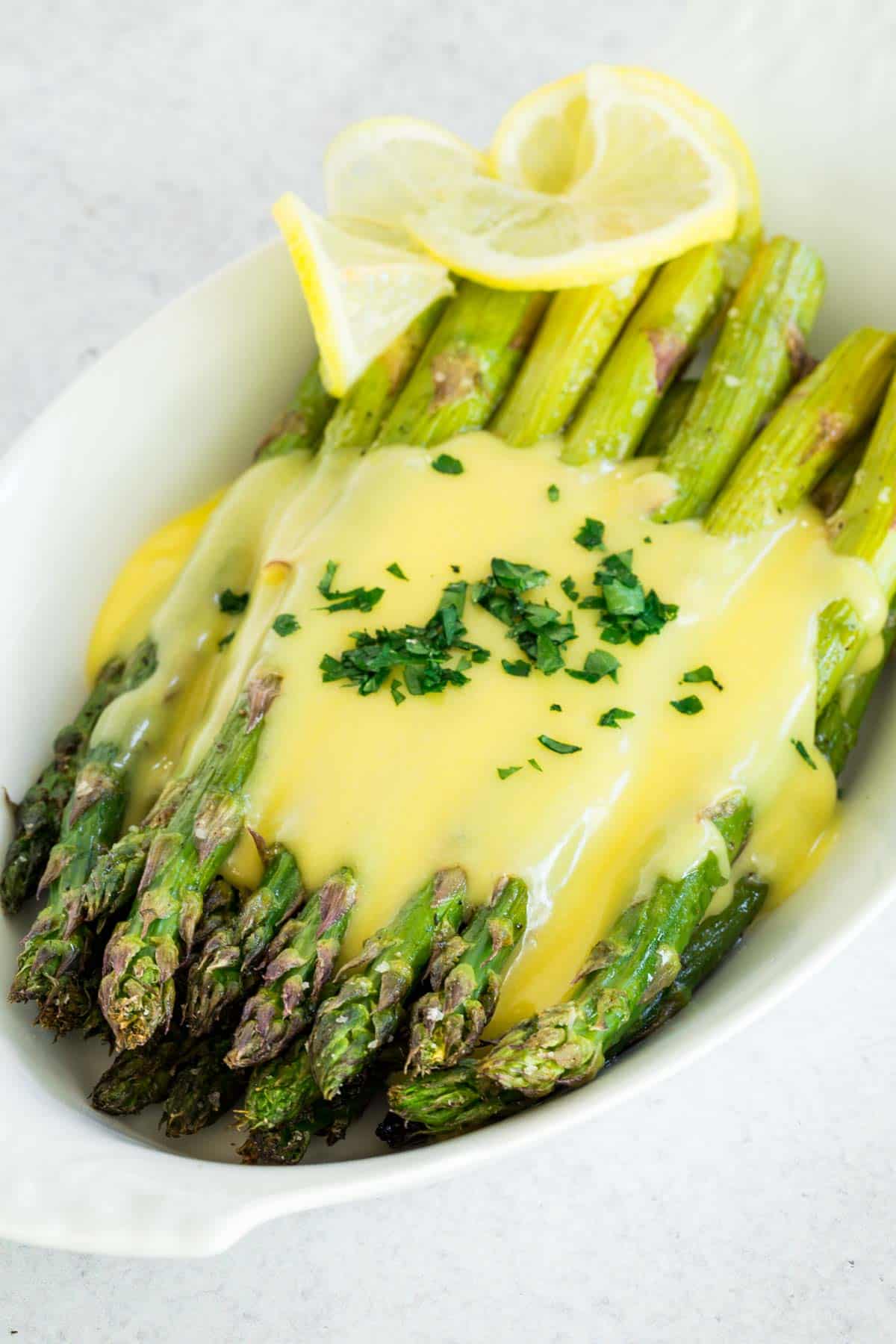The indoor photograph captures a professionally-arranged plate of asparagus set on a light gray table or countertop with darker gray stone-like lines. The rectangular image, approximately 5 inches high and 3 inches wide, features a white oval dish with a small lip handle visible on the lower left. The dish is brimming with about 20 pencil-length, relatively thick asparagus spears, transitioning from darker green at the lower left to yellow-green towards the upper right. These are topped with a generous drizzle of thick, creamy yellow hollandaise sauce, garnished with finely chopped green herbs, such as possibly cilantro or basil. Two lemon slices add a pop of brightness, enhancing the freshness and well-crafted appearance of the dish. The composition emphasizes the lusciousness and appeal of the food with detailed textures and vibrant colors, making the asparagus dish look both delicious and inviting.